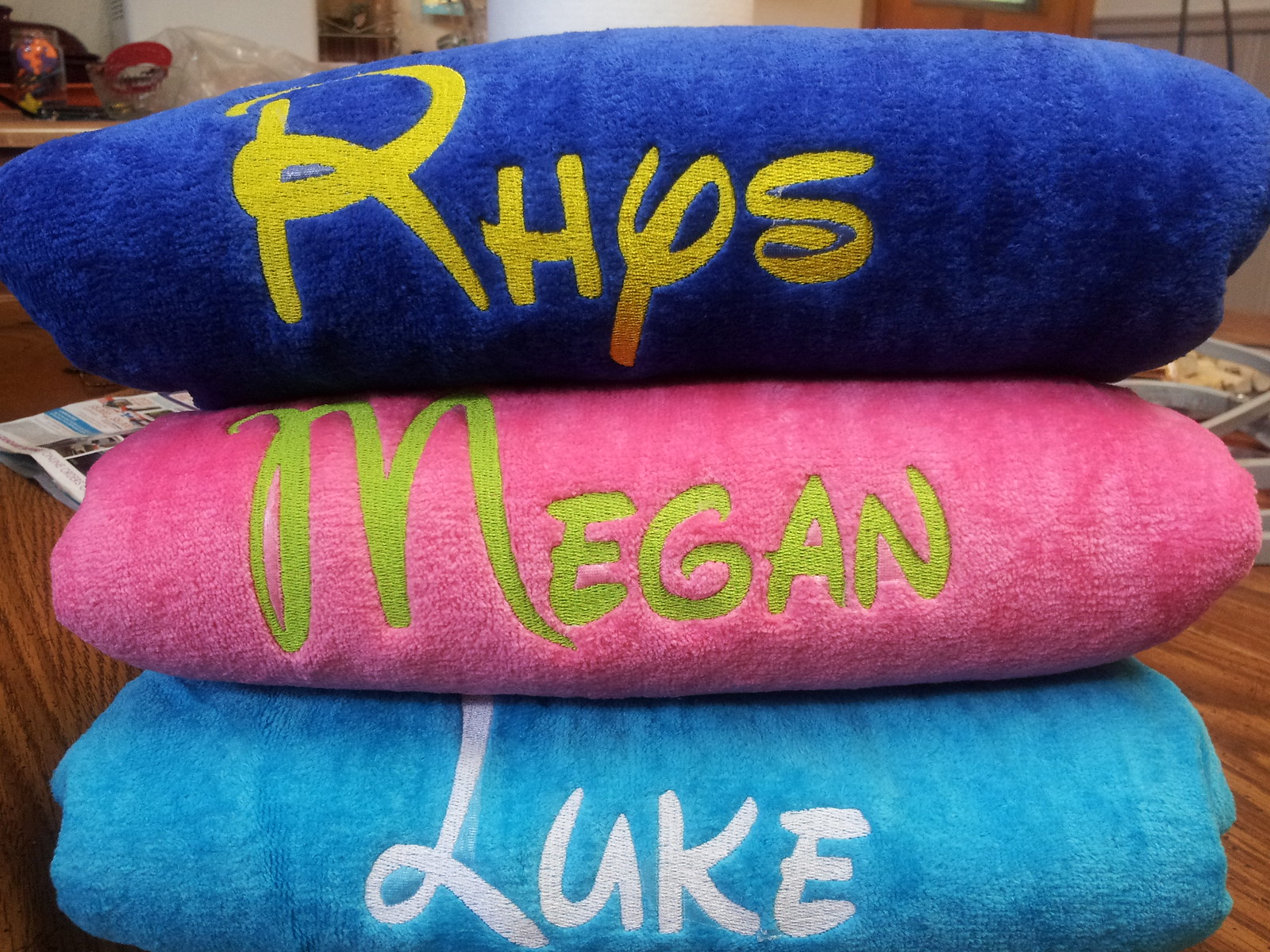The image depicts three neatly folded, monogrammed blankets stacked on a brown wooden table. The lowest blanket is a sky blue terrycloth featuring the name "Luke" in large, white, fun lettering. Above it, there's a pink blanket with the name "Megan" embroidered in vibrant green. Topping the stack is a royal dark blue blanket adorned with the name "Rhys" in a curly, whimsical script reminiscent of Disney lettering, rendered in a yellowish-gold thread. The scene is set indoors, evidenced by some debris and various items, such as magazines or books, scattered in the background.